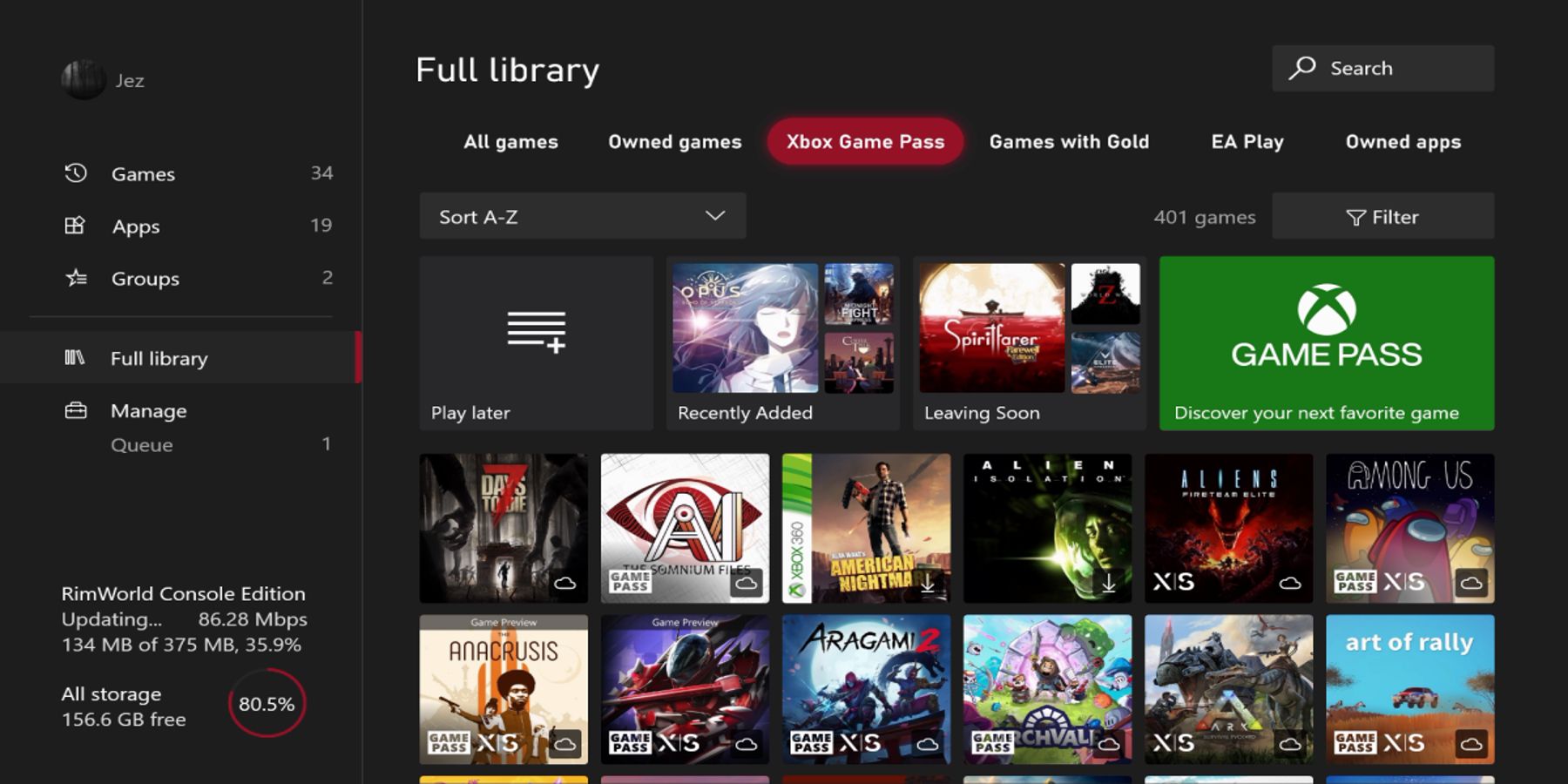The image depicts a detailed game launcher interface with a dual-pane layout. The left section of the interface features a vertical menu showing the user profile at the top, labeled "Jez." Below the profile section, there are categories for "Games," "Apps," and "Groups," listing counts of 34 games, 19 apps, and 2 groups, respectively. Beneath these categories, the menu continues with two additional items: "Full Library," which is highlighted, and "Manage." Due to "Full Library" being selected, the right section of the interface displays its corresponding details. 

In the right pane titled "Full Library," a horizontal menu presents various tabs including "All Games," "Owned Games," "Xbox," and "Game Pass." The "Game Pass" tab is currently active. Below this menu, sub-sections titled "Recently Added," "Leaving Soon," and "Play Later" are visible, providing organized access to the user's game collection and subscription details.